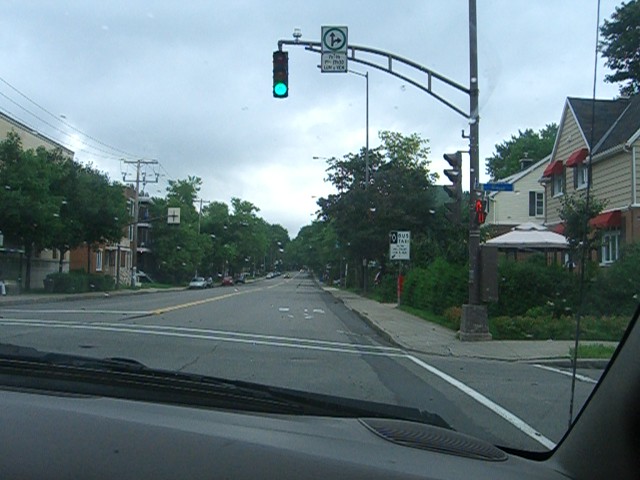The photograph captures a street scene from the perspective of the passenger seat on the right-hand side of a car, indicating a left-hand drive vehicle. The gray dashboard features a slightly darker gray speaker, and a windshield wiper rests against the bottom of the windshield with a thin black radio antenna extending upwards. The image has a vintage feel, likely from the 1990s or early 2000s, indicated by its grainy quality. The car is stopped at a T-intersection facing a traffic light that is green. Adjacent to the traffic light is a green-circled sign with arrows pointing straight and right. The intersection includes crosswalks marked with white lines. Surrounding the road are trees with green foliage and, to the right, a tan house with red awnings. In the distance, a brown metal pole supporting a silver arched pole stretches across the road, adding to the urban scenery. There are no text or time stamps on the photograph.